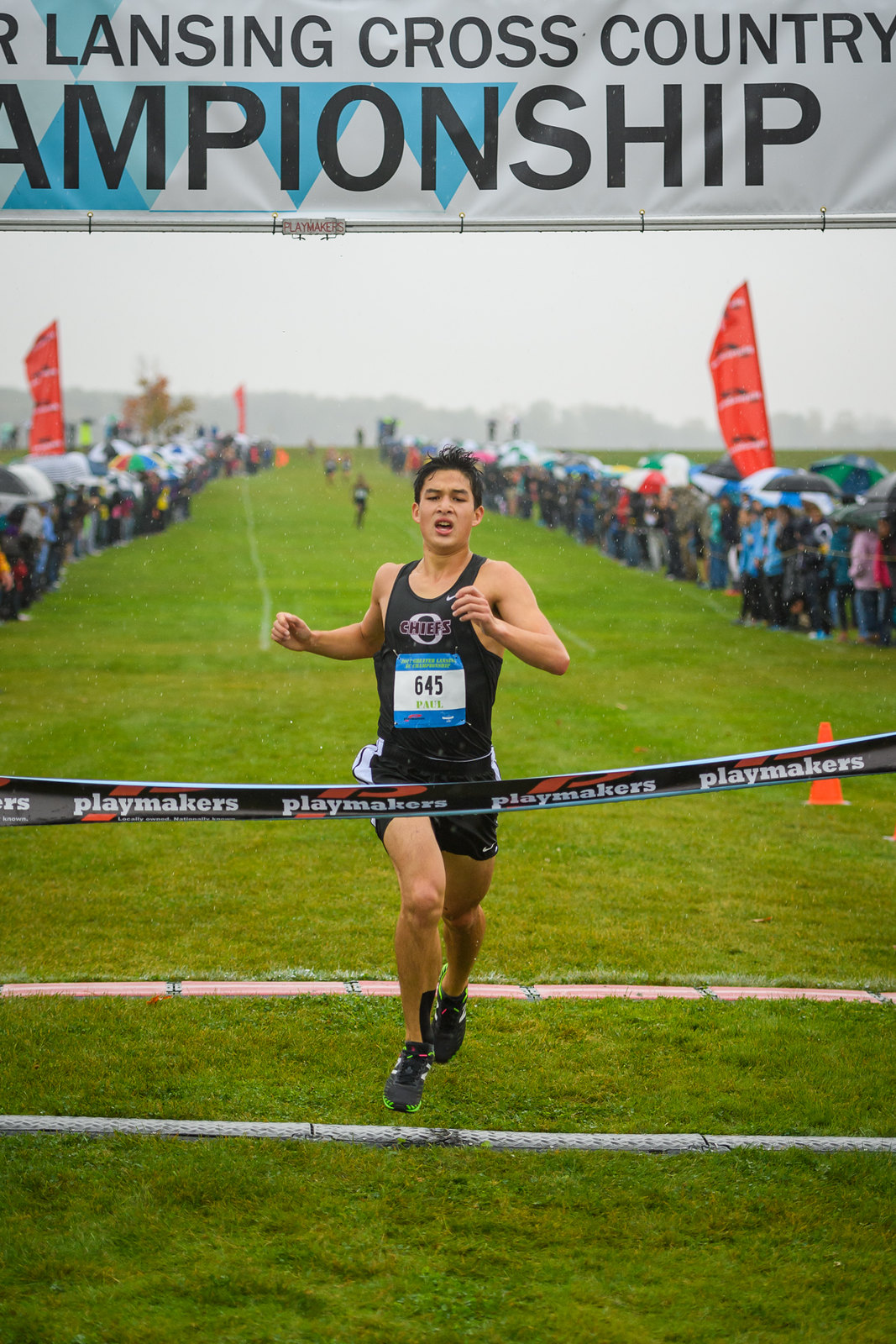In the image, we see a man crossing the finish line in a cross-country race at the Lansing Cross-Country Championship. The runner, an Asian male with short black hair and an open mouth, is wearing a black tank top with "Chiefs" emblazoned on it, black shorts, and black running shoes. His race tag reads "645 Paul". He is breaking through a recurring "Playmakers" banner with a yellow cone visible behind him. The scene takes place on a lush green grass field, flanked by spectators on either side, clad in various jackets and holding umbrellas due to the rain. The sky above is completely gray, with distant trees and blurred competitors visible, adding to the immersive atmosphere of the event.